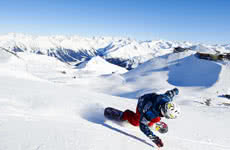In a stunning winter scene, a snowboarder clad in a distinctive blue long-sleeve coat, vibrant red pants, and a white helmet with yellow accents is captured in action. He skillfully maneuvers a curve on a snow-filled mountainside, with his black and colorfully detailed snowboard carving through the pristine white snow. His arms are extended for balance, revealing the black gloves he's wearing. The majestic background showcases mountainous terrain blanketed in snow, with intermittent patches of exposed mid-sections revealing rocky underlayers. Shadows play across the mountain slopes, creating a striking visual contrast. Above, the sky exhibits a beautiful gradient, transitioning from a light blue along the horizon to a deep, dark blue at the zenith. The scene is small, almost thumbnail-sized, yet it encapsulates the exhilarating essence of winter sports amid breathtaking natural beauty.